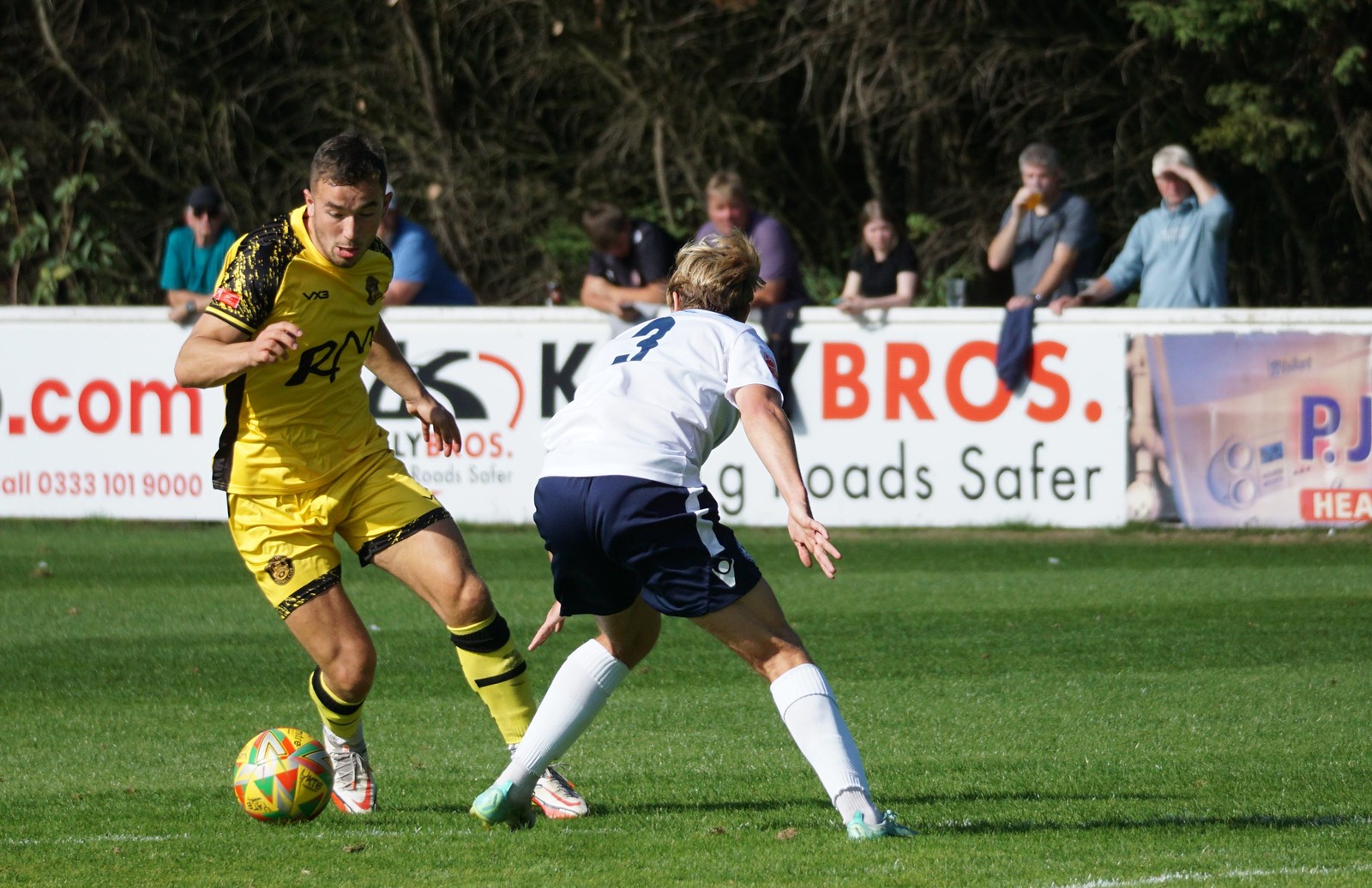The photograph captures an intense moment in a daytime soccer match played on a lush green field. In the foreground, two soccer players vie for control of a vibrant green, red, and yellow soccer ball. The player on the left, mid-kick, dons a distinctive white and black jersey with yellow shorts featuring black stripes and white-orange soccer cleats. His jersey appears to have the initials "RM" printed on the front. Opposing him, the player on the right, with his back to the camera, is bent forward, wearing a white jersey emblazoned with the number three, navy blue shorts, white knee-high socks, and white shoes. A white-railed fence adorned with various business banners stands in the mid-ground, showcasing partially visible names and logos with words like ".com," "bros," and "pads." Leaning on the fence are numerous spectators eagerly watching the action unfold. The backdrop features a thick tree line, stark and barren with many trees missing their branches and leaves, casting a sharp contrast against the vibrant scene on the field.